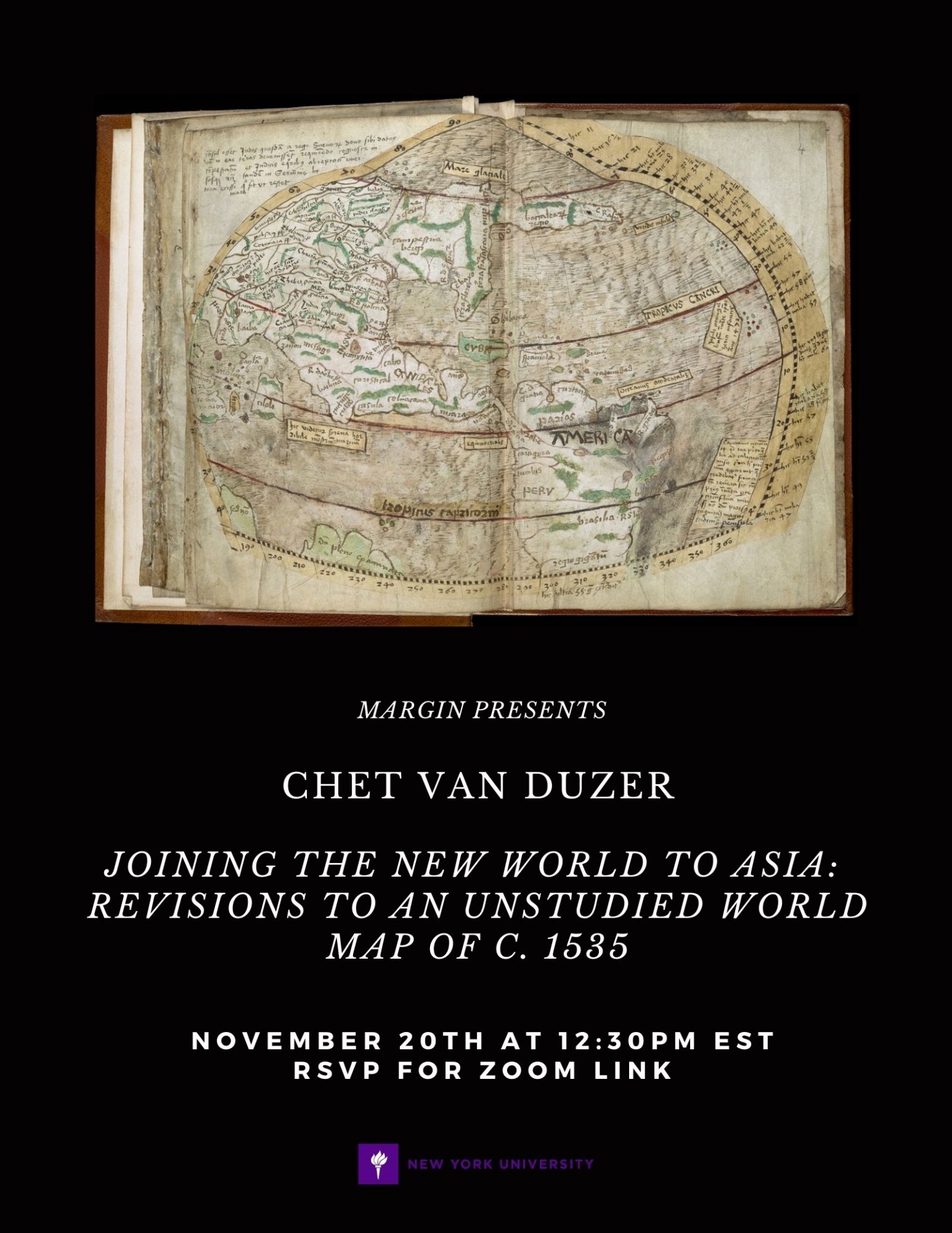The image is a flyer advertisement for a Zoom meeting hosted by New York University. The background is black, prominently featuring an aged, hand-drawn map from 1535, which illustrates a rough outline of North America, Mexico, Central America, and South America as they were perceived at the time. Above the map, the flyer reads: "Texas's Martin Presents, Chet Van Duzer: Joining the New World to Asia, Revisions to an Unstated World, Map of 1535." Below, in smaller text, it states: "November 20th at 12:30 PM EST, RSVP for Zoom Link." At the very bottom, within a purple box, is the New York University logo, accompanied by a square filled with purple containing a white torch symbol.